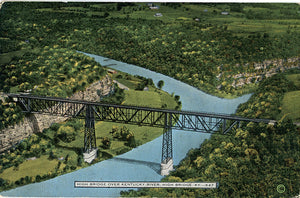This is a detailed depiction of a bridge over a river, likely a digital representation from a video game or an older image. The bridge is a brown, metallic trellis structure, possibly made of steel or iron, and appears to be designated for trains, as there are no visible roads. The bridge spans two pieces of land, supported by two posts; one stands on the grassy land, while the other emerges from the river. The calm blue river underneath splits into two sections, surrounded by lush, green vegetation on both sides and extending into the distance. A light brown, rocky ridge is visible on the left side, with grass that appears to be either inhabited or planted. The background is filled with green and some yellow-topped trees, indicating a clear weather setting. A small white text box with black writing is present at the bottom of the image, yet too small to decipher clearly, but it likely labels the scene as "bridge over Kentucky River."